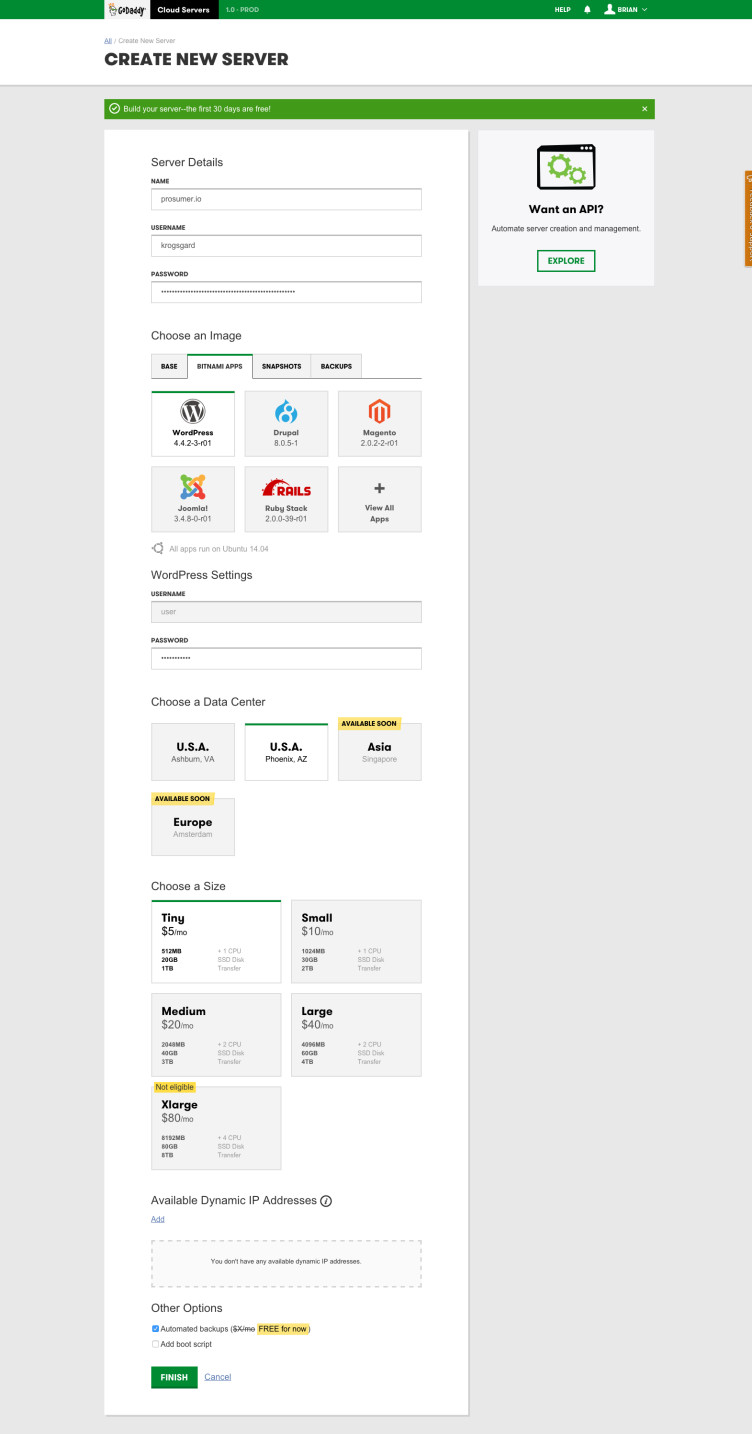The image showcases a website with a structured interface designed for server management. At the top of the page, there is a green banner featuring a white background with the text "GoDaddy" emblazoned in black. Below this, a sleek black banner with white text declares "Cloud Servers." 

On the right side of the header, the site offers quick access to "Help," accompanied by an icon of a bell and a user avatar—a white silhouette of a person from the shoulders up labeled "BRIAN" in capital letters.

As you scroll down, the first section features a prominent call-to-action button with a white background and large black text stating "Create New Server." This section is followed by another banner with a green header that reads "Build Your Server — the first 30 days are free." 

In the main body of the page, details about the server configuration are displayed on a white background. It includes fields for server name, username, and password, all pre-populated for convenience.

To the right of these fields, there is a section beginning with a small square, containing a black square at the top housing two green gears. This section provides information about API options for automating server creation and management, labeled "Want an API?" and features a blue button encircled by a greenish-blue border that says "Explore."

Further down, the page offers options to "Choose an Image," including "Base," "Bitnami Apps," "Snapshots," and "Backups." Additional settings sections include "WordPress Settings," "Choose a Data Center," "Store," "Choose a Size," and "Available Dynamic IP Addresses," ending with a segment titled "Other Options."